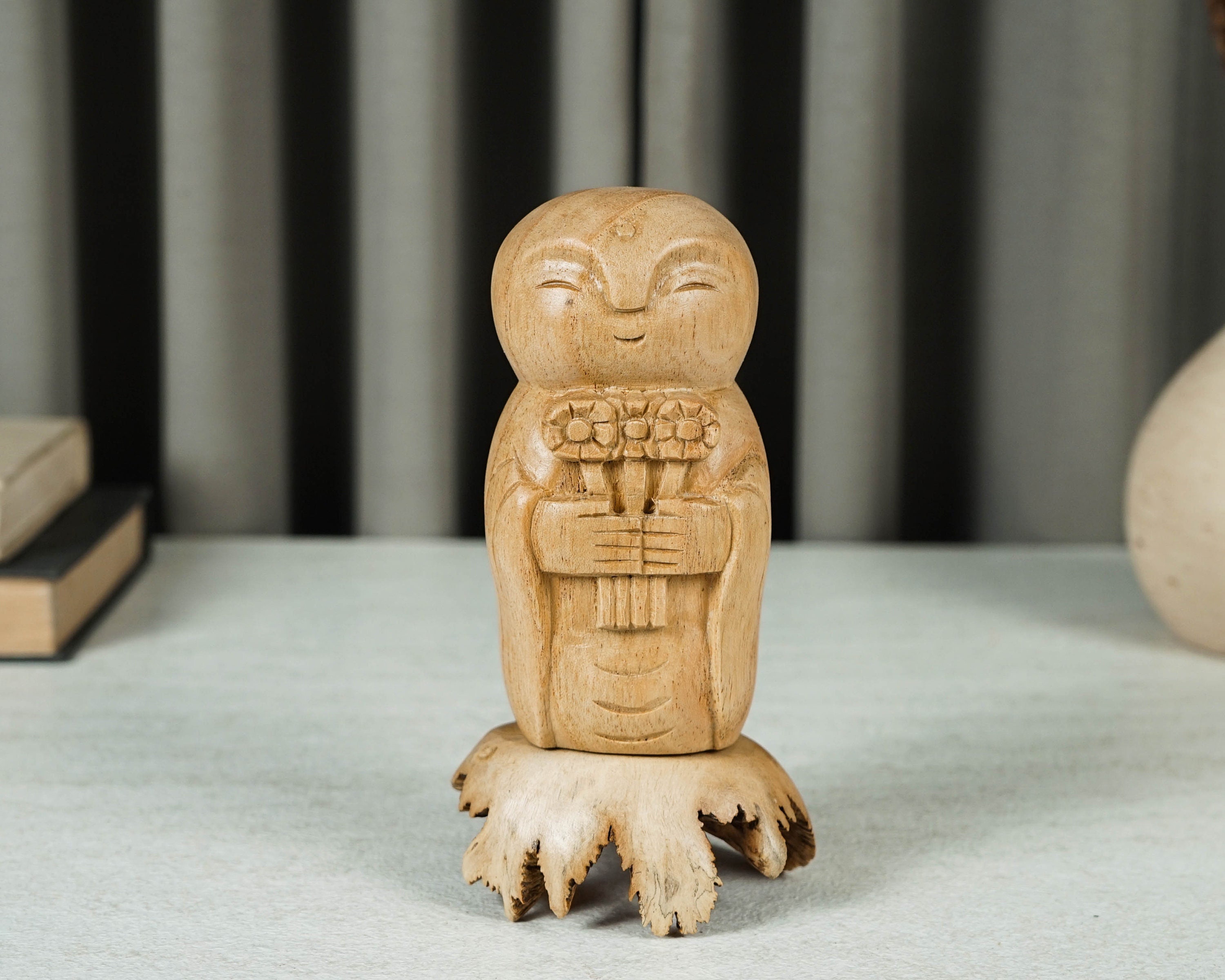This well-lit indoor photo showcases a meticulously carved statue, carved from light tan wood, exuding a happy and serene aura. The statue resembles a cheerful, bald man with a round face, closed eyes, and a gentle grin, giving off a peaceful and joyful vibe. Draped in a long, flowing robe that cloaks its rectangular yet slightly curved body, the statue brings intricate craftsmanship to life. The figure's hands are delicately brought together over its tummy, holding three flowers with four stems, each bloom featuring round centers surrounded by square petals. The statue is propped up by a base that appears to be shaped like carved leaves, adding a naturalistic touch with a subtle shine. Positioned on a grey or white surface, the scene is elegantly set against a backdrop featuring two stacked books in black and white, and a geometrical circular object. The setting is further enriched by grey curtains or vertical blinds, enhancing the professional, polished look—ideal for product showcasing. The image boasts clear pixels and pristine lighting, accentuating the fine details and serene beauty of the wooden statue.